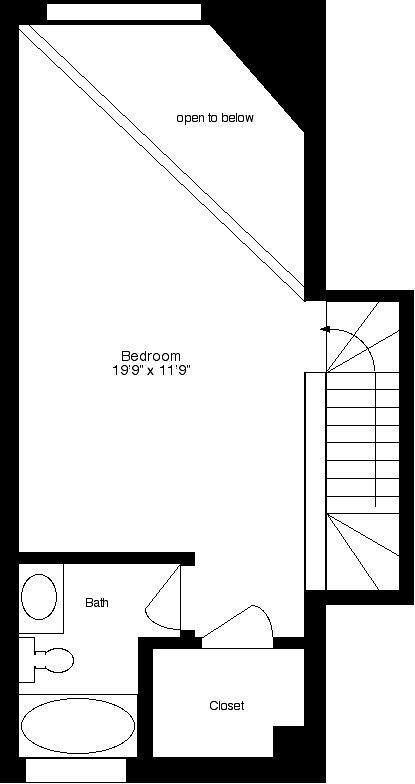The image showcases floor plans for a section of the house. The plans are outlined with a very thick black border. Towards the right side of the plan, there's a prominent extension that seems to represent a stairwell or an open space with a large opening labeled "Open to Below" in the upper right corner. Two light blue lines span across this space, indicating structural features or boundaries.

In the central area, there's a spacious bedroom dimensioned at 19'9" by 11'9", with an entrance doorway. Attached to the bedroom is a bathroom, clearly depicting the sink, toilet, and bathtub. The bedroom also features another doorway and an exceptionally large closet, emphasizing the expansive nature of the room. Additionally, there's an area with what appears to be a door leading out towards the stairwell, all contained within the thick black border of the plan.